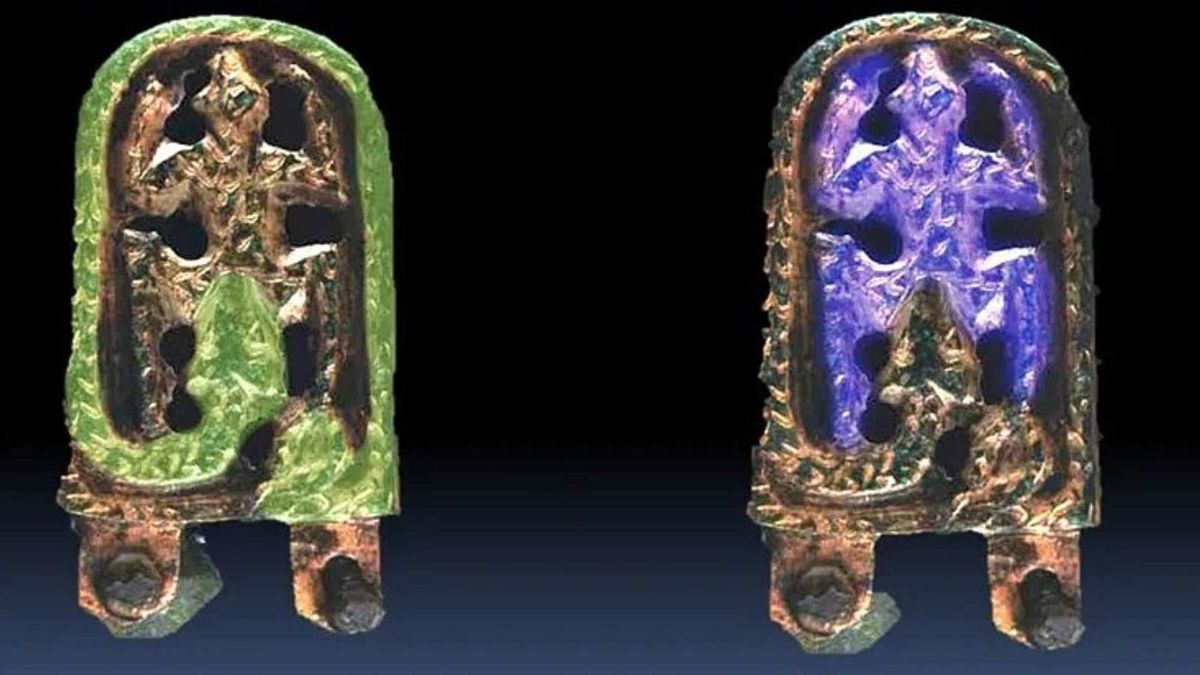The image depicts two ancient-looking artifacts that seem to be related to jewelry or possibly religious symbols. Both artifacts are identical in shape and structure: they are oval at the top and taper down to a flat bottom, where two rusted metal attachments with holes are visible, likely for bolts to secure them in place.

Each artifact features a serpent coiled around a human figure. The serpent's head is positioned near the crotch of the spread-eagle human figure, whose arms are raised and legs are extended downward. The artifact on the left has a serpent that appears to be an emerald green, while the human figure is colored in a vibrant lime green with green jewels. The artifact on the right showcases a metal serpent, possibly once gold-plated, encircling a purple gem-bodied figure. The serpent and human figures give the impression of Mesoamerican art, emphasizing the snake's symbolic significance.

Both pieces have slightly rusted features, suggesting their ancient origin or archaeological significance. The artifacts are displayed against a black background, which may indicate they have been digitally placed for detailed examination.